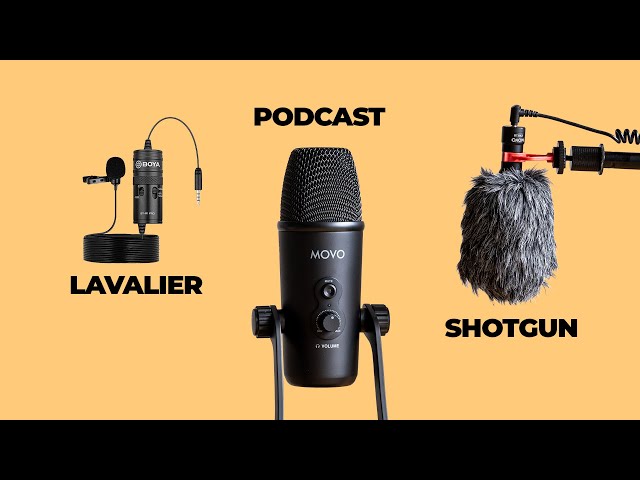This instructional photograph showcases three types of microphones against a mustard orange background, with black lines bordering the top and bottom. On the left, labeled "LAVALIER" in black letters, a small, black gumdrop-sized microphone is displayed. It rests on a circular stand and includes a battery pack and an attached jack cord. In the center, prominently displayed, is a podcast microphone labeled "PODCAST" above it. This cylindrical microphone, approximately six to eight inches long, features a metal mesh top and two tuning knobs, likely for power and volume, set into its black base. The brand "Movo" is visible on the microphone, which is held upright on a grommet stand, secured by screws for adjustable positioning. On the right side, labeled "SHOTGUN," the photograph shows a large, fuzzy shotgun microphone, typical in filmmaking, mounted on the tip of a black boom. This microphone has a felt wind or breath guard, emphasizing its use in capturing high-quality audio while minimizing ambient noise.